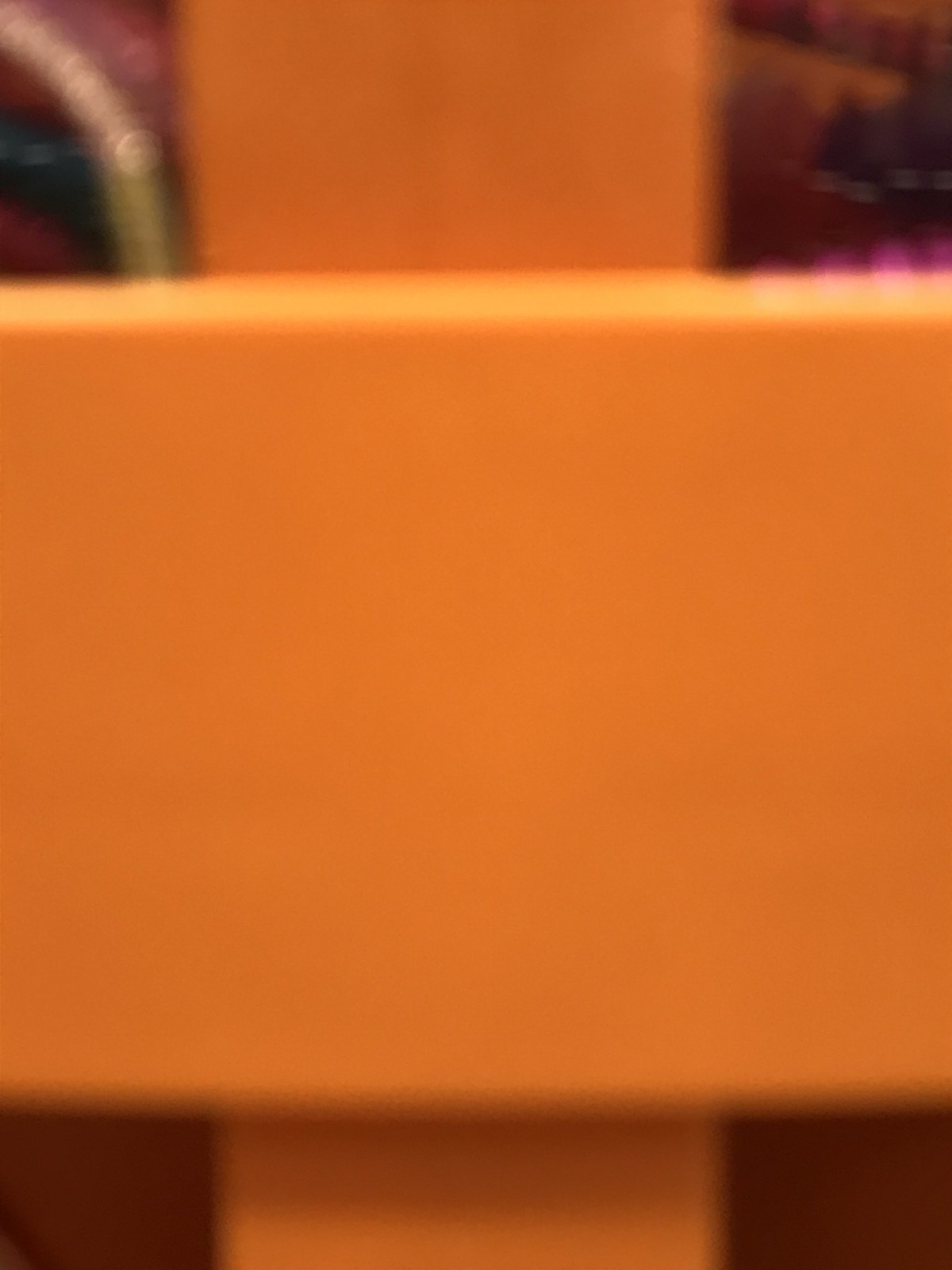This photograph appears to be an abstract image dominated by warm colors and an intriguing composition. The picture is somewhat blurry, making it challenging to discern precise details, yet it offers a blend of dark orange, light orange, and maroon or wine tones that create a visually captivating palette. Prominently featured are two overlapping orange shapes forming a cross-like pattern. The horizontal piece is broad and spans across the majority of the image, while the vertical segment is slightly narrower but equally intense in its vibrant orange hue. In the upper left corner, a curved silver element adds a contrasting metallic touch to the overall warm composition.